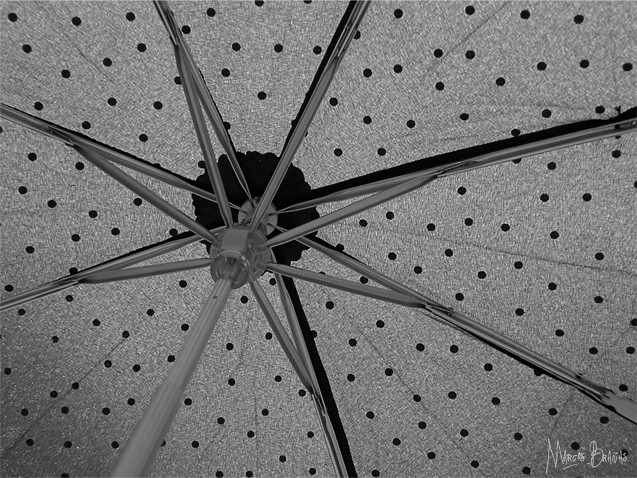This is an artistic rendering—possibly a high-quality drawing or a photograph—depicting the inside view of an umbrella. The image focuses on the metal spokes radiating from the central handle. The umbrella's covering is a light gray with evenly scattered black polka dots, all viewed from beneath. The black and white composition accentuates the structural details of the umbrella's framework. In the bottom right corner, there is a signature in faint, cursive white that appears to read "Marcus Bellino," although the last name is somewhat difficult to decipher. This unique perspective highlights the symmetric beauty and intricate design of the underside of the umbrella.